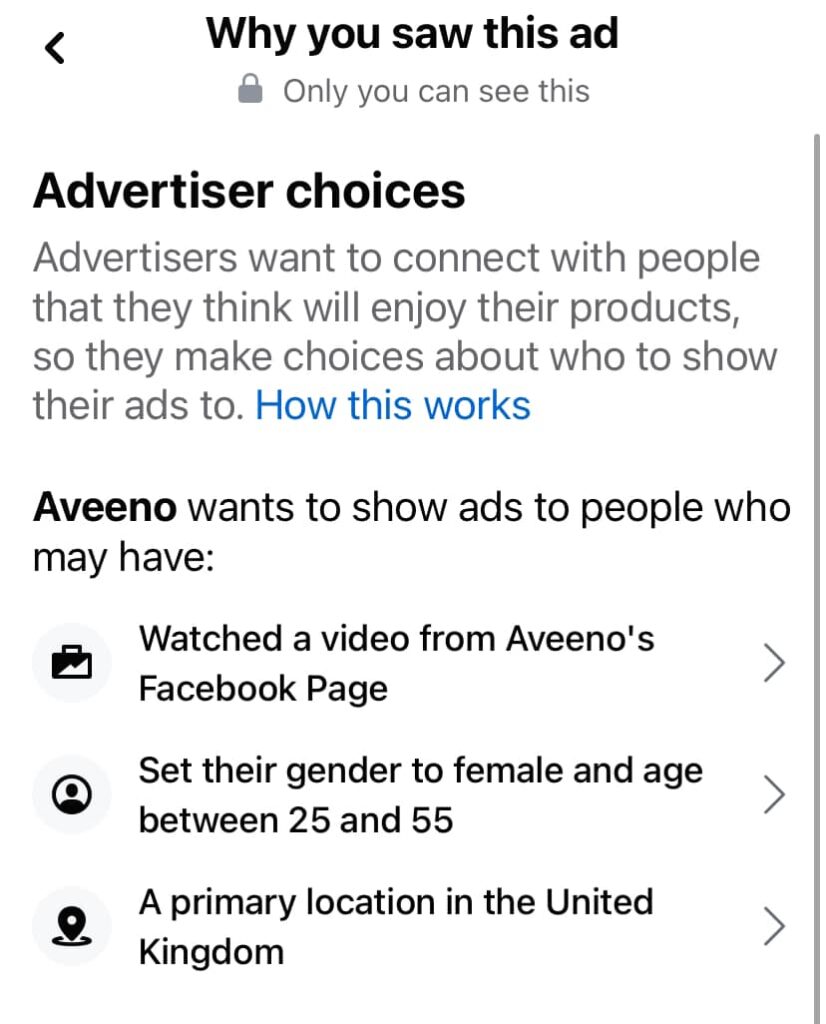The image depicts a screenshot from a user's encounter with an advertisement option. 

In the top left corner, there is a back arrow, allowing users to return to the previous screen. Centrally positioned at the top are the words "Why you saw this ad." Directly below this text is a lock icon accompanied by grey text stating "Only you can see this," ensuring privacy for the user. 

The main title, "Advertiser Choices," is displayed prominently in bold black font. Beneath it, a grey subtitle explains, "Advertisers want to connect with people that they think will enjoy their products, so they make choices about who to show their ads to." To the right of this explanatory text is a blue hyperlink labeled "how this works," inviting users to learn more about the ad targeting process.

Further down, the advertiser "Aveeno" is mentioned in bold text, indicating their intent to show ads to a specific audience. Aveeno has targeted individuals based on three criteria:

1. **Interest in Aveeno's Content** - Individuals who have watched a video from Aveeno’s Facebook page, accompanied by an icon that appears to represent a briefcase or video.
   
2. **Demographic Information** - Users who have set their gender to female and are aged between 25 and 55. This information is indicated with a blank profile picture icon on the left.
   
3. **Geographic Location** - Users whose primary location is in the United Kingdom, symbolized by a location icon.

Aligned to the right of these criteria are rightward-facing arrows, suggesting that users can interact with these options for further details or actions.